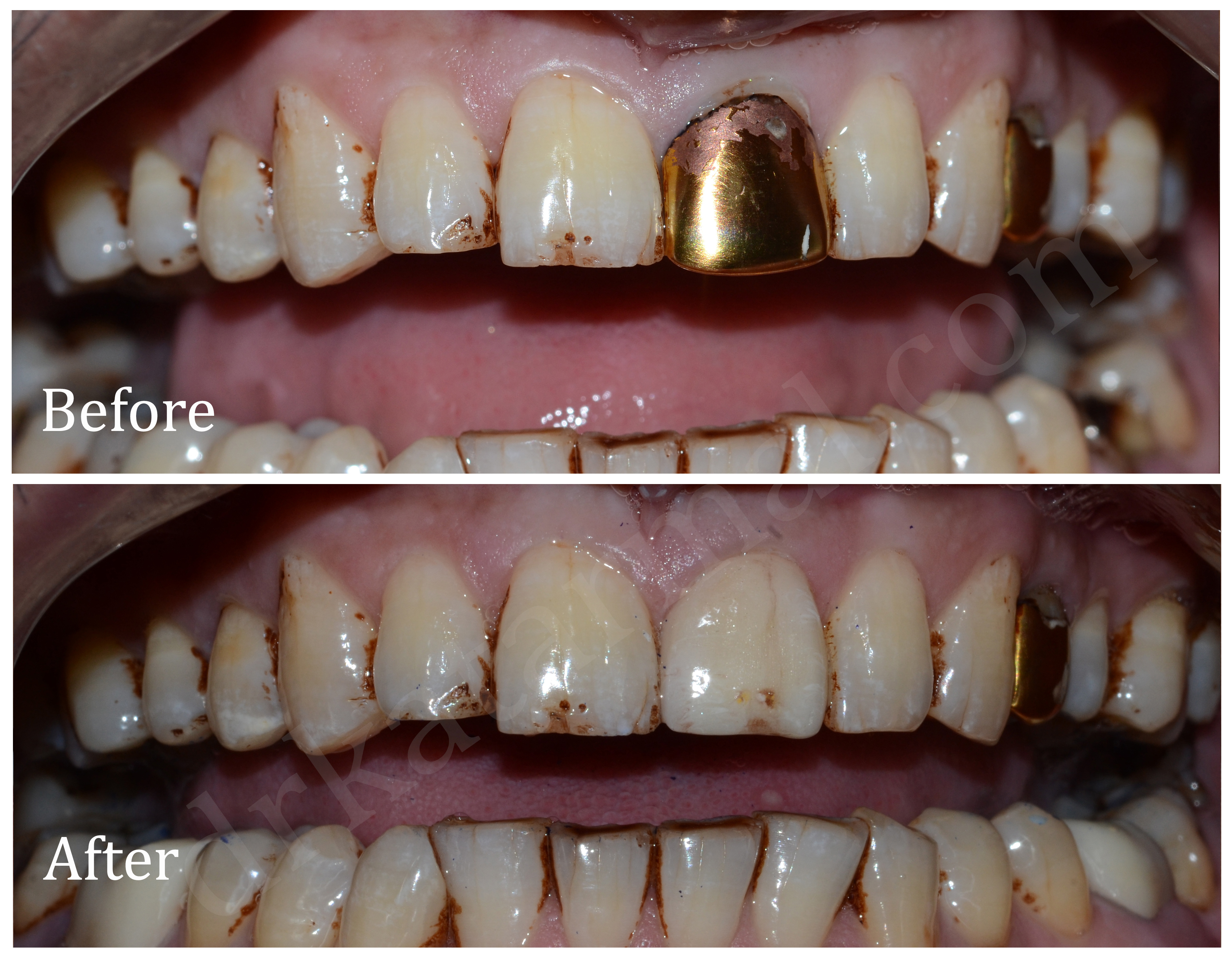This composite image showcases a before-and-after sequence of a dental procedure on a person's teeth, appearing reminiscent of a medical textbook or advertisement. The "before" image presents the upper and lower rows of teeth, where the focus is notably on the top front left tooth with a conspicuous golden cap. The rest of the teeth display signs of discoloration and misalignment, with some described as having a rusty hue. The surrounding gum line near the gold-capped tooth appears white in contrast to the other gums.

In the "after" image, the gold cap on the top front left tooth has been removed and replaced with a white tooth, likely a porcelain crown, restoring uniformity to the patient's smile. The gum line, previously white near the golden tooth, now matches the healthy pink color of the surrounding gums. The transformation highlights the improved appearance and condition of the teeth and gums following the dental intervention, suggesting advancements in dental restoration techniques.